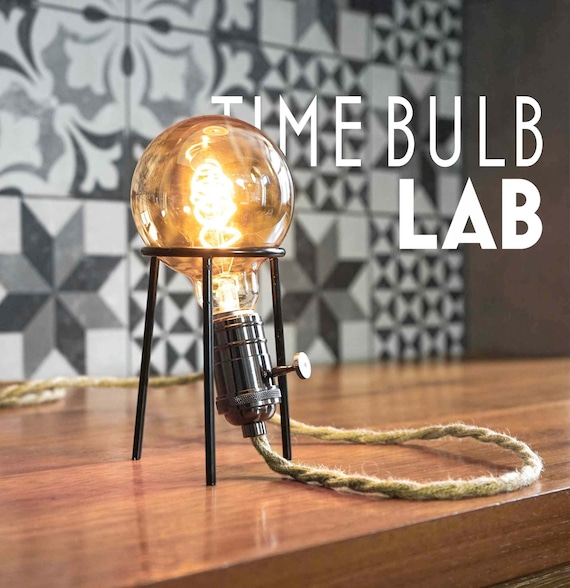The image displays a lit, vintage-style light bulb with a visible coiled filament, set on a small tripod-like black metal stand. The stand features a circular holder around the bulb and a twist knob resembling a nail head for turning the light on and off. The light bulb, exuding a reddish glow, is connected to a twine-like, fabric-coated brown electric cord that trails off into the background.

This setup rests on a polished wooden desk, creating a warm, inviting atmosphere. The background is decorated with an abstract pattern of black, white, and gray tiles, including designs such as eight-pointed stars, hourglass shapes, and flowers composed of parallelograms and triangles facing various directions. Overlaying this backdrop, partially obscured by the light bulb, are the bold white words "Time Bulb Lab," with some letters partially hidden behind the bulb, adding a modern touch to the vintage aesthetic.